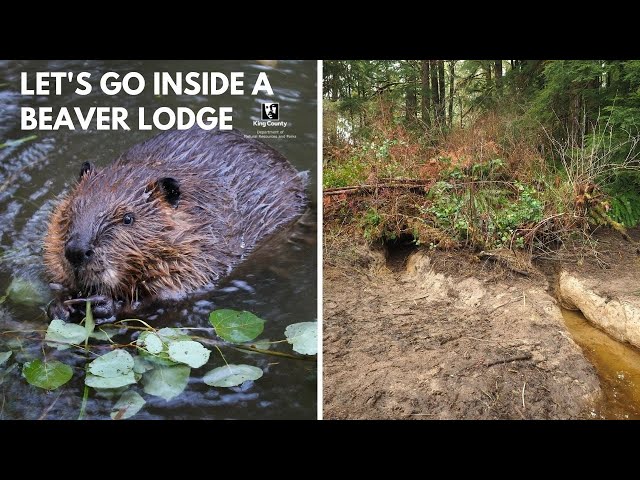The image features two distinct photographs, presented side-by-side with a black border on the top and bottom, possibly as a thumbnail for a YouTube video or part of a presentation or flyer. 

The photograph on the left shows a beaver partially submerged in water, its brown fur appearing wet with a tan area around its face. The beaver is angled towards the bottom left corner and is holding a small cluster of leaves. Above this image, there is white text that reads, "Let's go inside a beaver lodge."

The photograph on the right captures what is presumed to be the beaver's lodge. It showcases a forested area with a dirt embankment, where a dark, deep hole—likely the entrance to the lodge—is visible. Tall grass and branches surround the lodge, with a creek or water body nearby, suggesting an intricate habitat within a wooded ecosystem. The background includes more trees, adding to the sense of a natural, undisturbed environment.